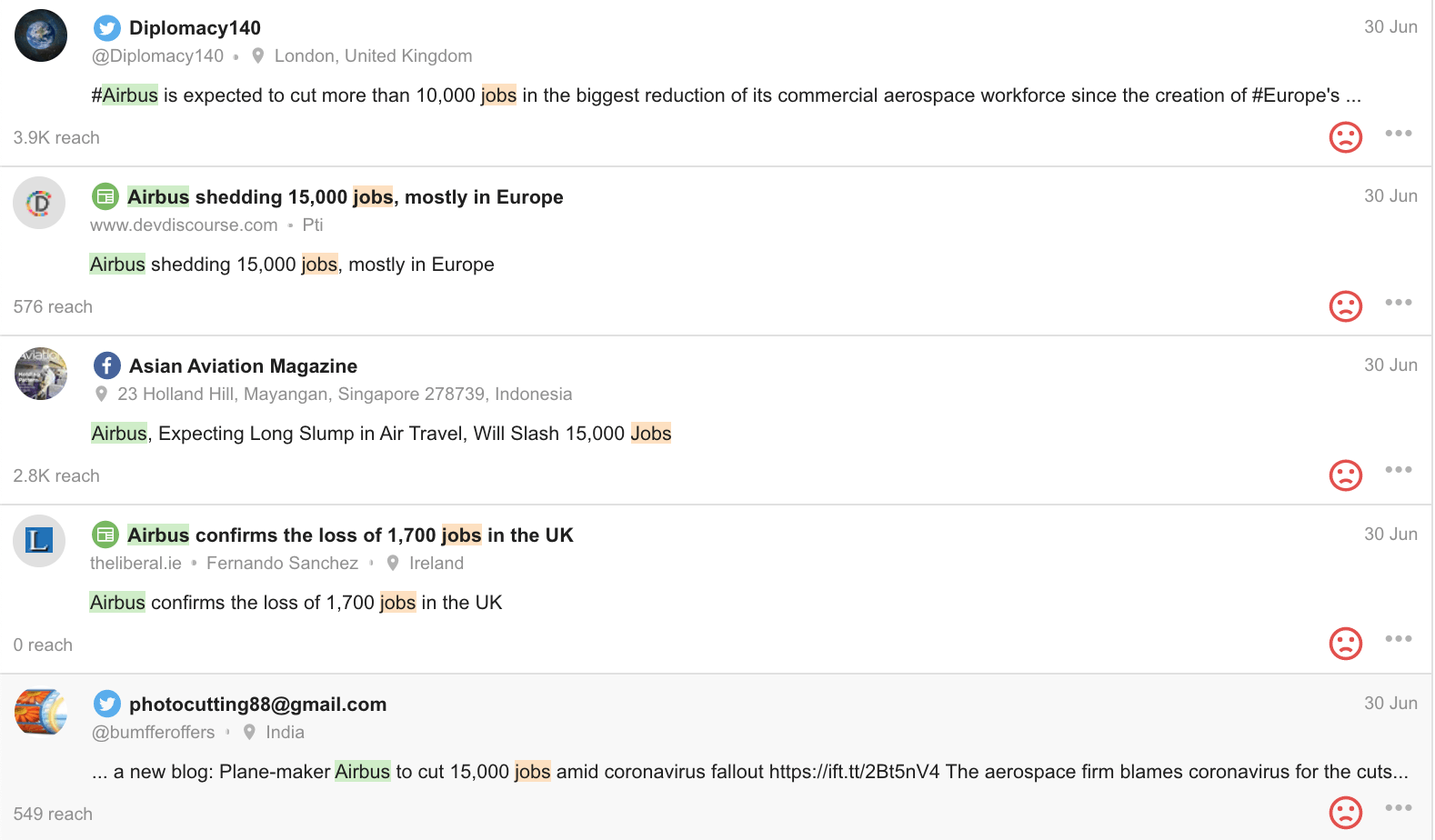In this image, at the top left corner, the username "Diplomacy 140" is displayed alongside a Twitter icon. Directly below, the handle "@Diplomacy140" and a pin location icon indicate the user is from London, United Kingdom. The user has posted a comment using the hashtag "#Airbus," stating, "Airbus is expected to cut more than 10,000 jobs in the biggest reduction of its commercial aerospace workforce since the creation of Europe."

Beneath this, the comment section starts with a remark about "Airbus shedding 15,000 jobs, mostly in Europe." Following this, there's a Facebook icon next to "Asian Aviation Magazine," which comments, "Airbus expecting long slump in air travel, will slash 15,000 jobs."

Continuing down, another comment mentions, "Airbus confirms the loss of 1,700 jobs in the UK." At the very bottom left of the image, we see a Twitter icon near the name "photocutting88@gmail.com" with a comment, "New blog: Planemaker Airbus to cut 15,000 jobs amid coronavirus fallout."